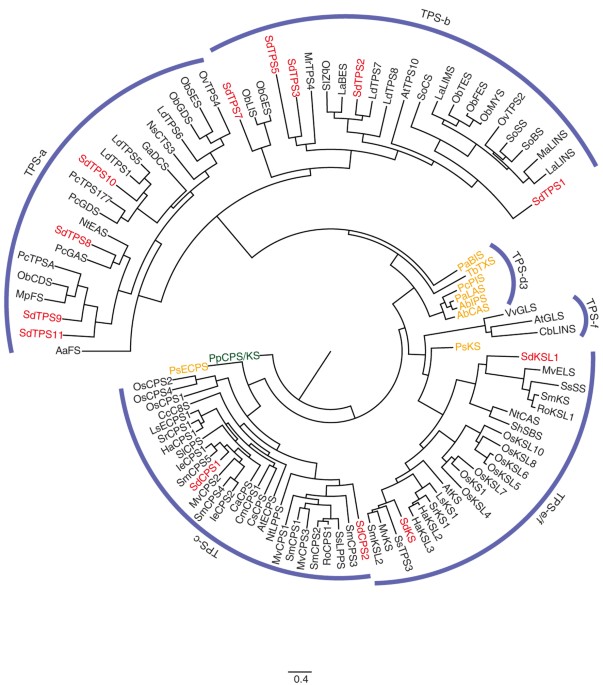This image is a detailed diagram exhibiting a complex network of pathways and directions, segmented into four quadrants. Each quadrant is labeled with identifiers: TPS-A, TPS-B, TPS-C, and TPS-E/F. The quadrants feature numerous codes and text elements in varying colors—black, red, yellow, and occasionally green—illustrating connections and flows. Blue, semicircular arcs of information at the top of each segment accentuate the pathways, bringing a coherent visual structure to the diagram. The pathways, depicted as lines and curves with intersecting brackets, indicate relationships and sequences among the labeled components, radiating outward from the center, resembling a structured scientific notification system.